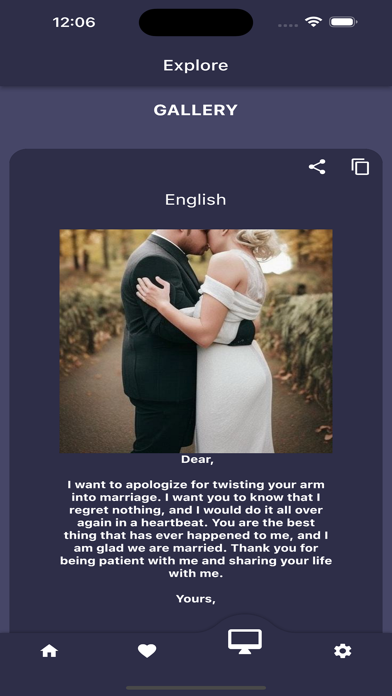This image is a screenshot from a phone displaying an app interface with a dark blue background. At the very top of the screen, the time is displayed as 12:06, followed by a central black oblong circle, the Wi-Fi signal icon, and a full battery icon. Below this, in bold white font, the word "Explore" is prominently featured.

Just beneath "Explore," there is a lighter blue navigation bar labeled "Gallery." Following this, a darker blue box appears with a series of navigational icons including a link, a small half-triangle, and a stack of boxes that suggest the presence of additional images, all located in the top left corner of the box.

Prominently in the center of the screen, the word "English" is displayed. Directly below, there is a photograph of a bride and groom dancing along a path lined with bushes. The scene appears to be set in an autumn forest, as yellow leaves adorn the surrounding trees, enhancing the romantic atmosphere.

Beneath the photo, text in white font reads: "Dear, I want to apologize for twisting your arm into marriage. I want you to know that I regret nothing and I would do it all over again in a heartbeat. You are the best thing that has ever happened to me, and I am glad we are married. Thank you for being patient with me and sharing your life with me, Yours."

At the very bottom of the screen, a row of icons is displayed: a home button, a heart button, a computer screen button, and a settings button.